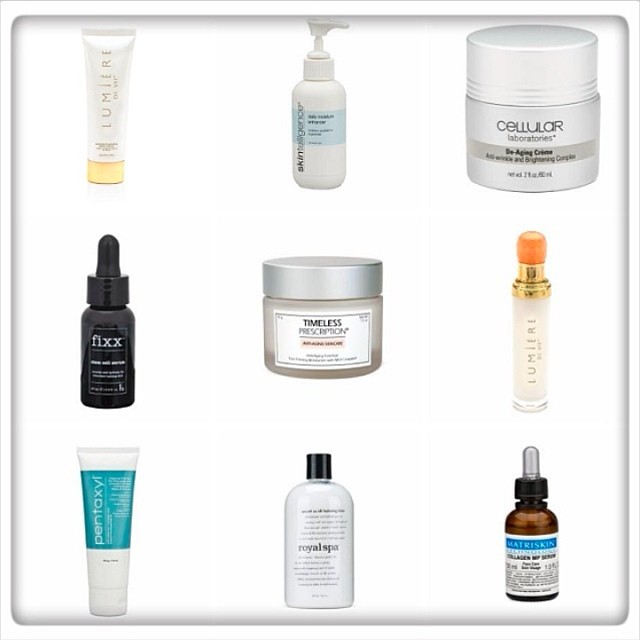Here is a cleaned-up and detailed caption for the image:

"This image showcases a bundle of nine beauty and skincare products arranged in a three-by-three grid, set against a clean white background. Each product is enclosed within a tile that has a subtle gray gradient and border radius, giving the overall presentation a polished, web-friendly look.

- **Top Left**: A white squeeze bottle labeled 'Lumiere' with a distinctive golden cap at the base.
- **Top Center**: A soap dispenser-style bottle, partially obscured, branded 'Skin Something'.
- **Top Right**: A beauty product bottle labeled 'Cellular Laboratories Anti-Aging Cream'.
- **Mid Left**: A sleek black droplet bottle from the brand 'Fixx'.
- **Center**: A blurry beauty product bottle labeled 'Timeless Prescription Skin Care'.
- **Mid Right**: Another elegant bottle labeled 'Lumiere'.
- **Bottom Left**: A squeeze bottle with the brand 'Pentoxyl'.
- **Bottom Center**: A wider bottle branded 'Royal Spa'.
- **Bottom Right**: A droplet bottle reading 'Matris Skin'.

Each product in this assortment appears to be part of a curated selection, ideal for a comprehensive skincare routine."